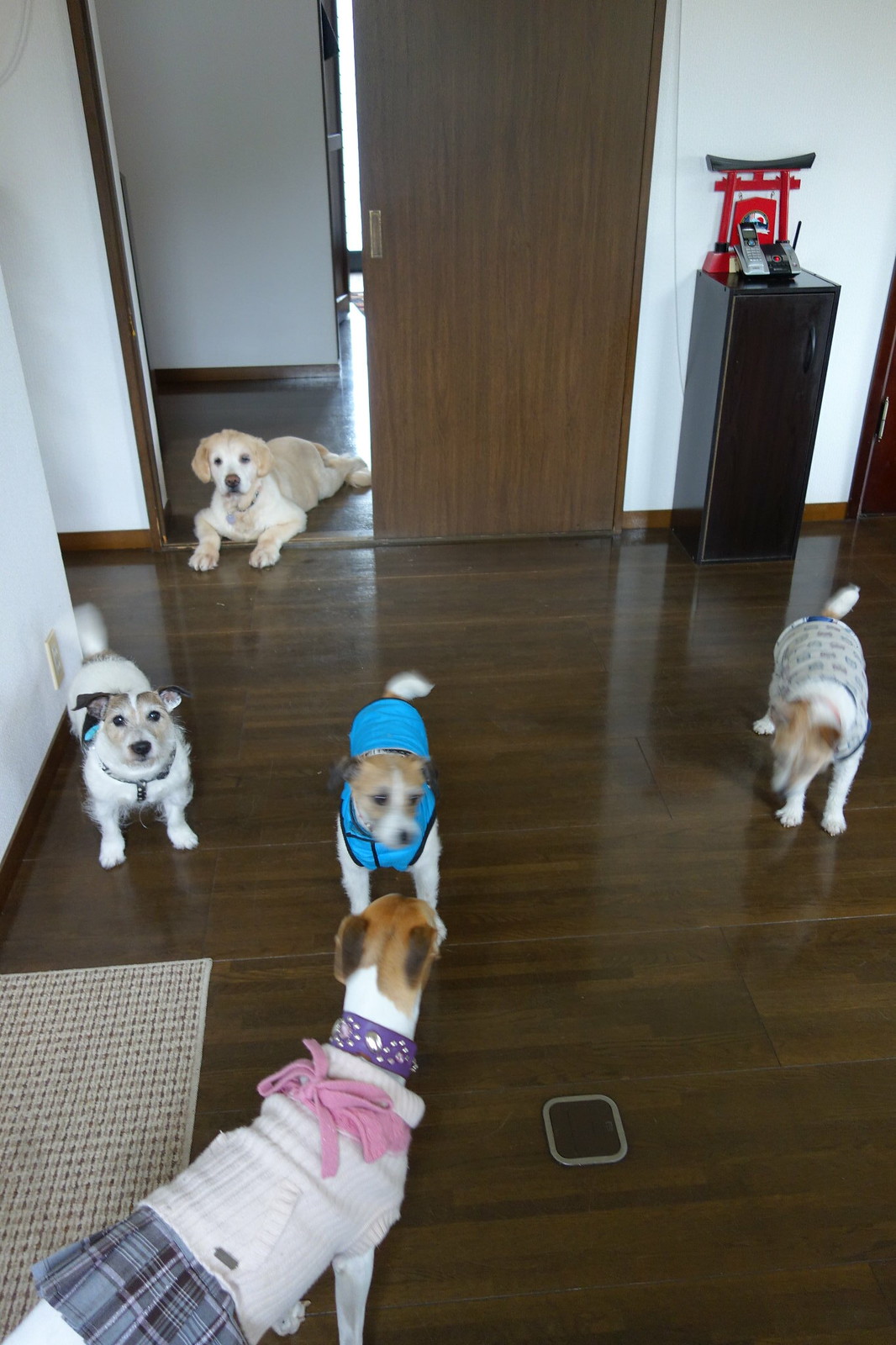The photograph depicts the interior of a house with polished brown hardwood floors. The focus is on five dogs, each adorably dressed in various doggie outfits. Dominating the background, an open brown wooden sliding door reveals an older, possibly a Labrador or golden retriever, relaxed with a big brown nose, sitting in the passageway of white plaster walls with brown skirting and door frames. In the main part of the room, to the left, a Jack Russell Terrier in a harness gazes directly at the camera. At the center, another Jack Russell Terrier, wearing a light blue coat, has a blurry face, indicating movement. On the right side, yet another Jack Russell in a coat confronts the center dog. Front and center, another slightly taller dog, clad in a warm white coat adorned with a pink bow and a purple studded collar, faces the middle Jack Russell. The cozy room features a dark wooden floor, a small table with a telephone, and a depiction of what looks like an oriental or Shinto temple, with the dogs milling around in their outfits, contributing to the charming chaos.